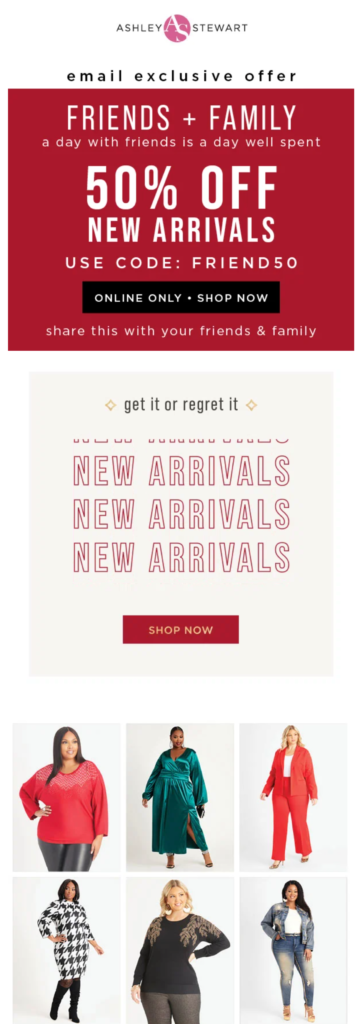**Caption:**

Ashley Stewart Email Exclusive Offer - A Day with Friends is a Day Well Spent

This vibrant advertisement promotes an exclusive email offer from Ashley Stewart, highlighting a generous 50% discount on new arrivals. It features the tagline, "A day with friends is a day well spent," encouraging shoppers to share the deal with friends and family. The ad showcases a diverse group of six confident plus-size women, modeling an array of stylish outfits ranging from formal wear to casual, outdoor attire. Set against a clean, off-white and cream-colored backdrop, the models radiate confidence and elegance, reflecting the brand's commitment to inclusivity and style. Below the main image, a smaller section urges viewers to "Get it or regret it," reinforcing the allure of the latest fashion arrivals. This online-only offer is a must-see for anyone looking to enhance their wardrobe with fashionable pieces from Ashley Stewart. Shop now and share the love with those close to you!